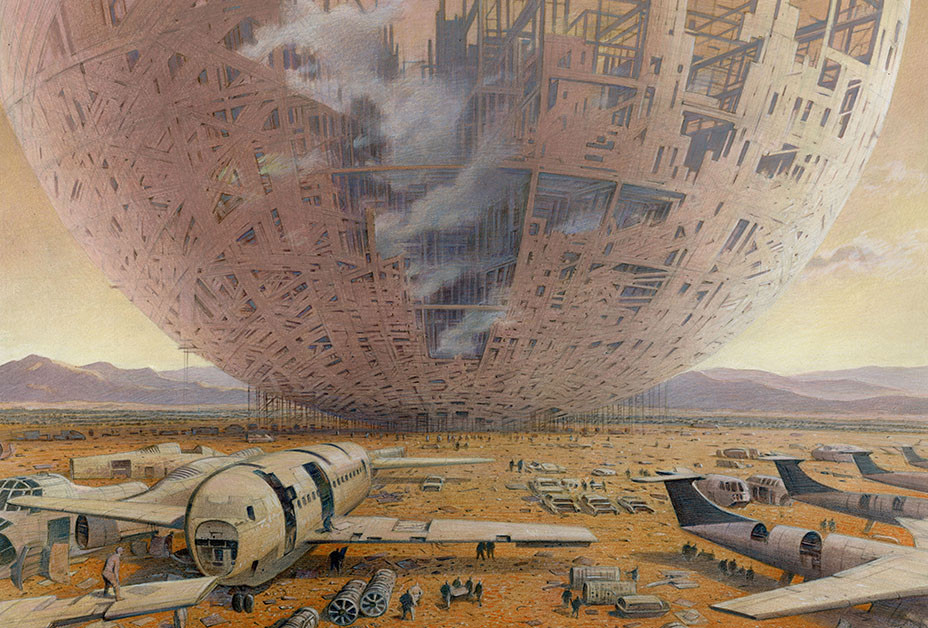This detailed, sci-fi illustration depicts a massive spherical structure, reminiscent of the Death Star, under construction. Rising from the horizon and towering beyond the sky, the sphere is composed of brown, scrap-like metal pieces, resembling intertwined steel I-beams or a giant rubber band ball. The scene unfolds over a vast, mustard-yellow desert landscape, bordered by mountains in the distance. In the foreground lies an expansive dirt field that resembles a salvage yard or airfield, cluttered with incomplete, old-school airplanes and their frames. These copper-red aircraft seem to be in the process of being constructed or disassembled by numerous people bustling about, carrying materials and parts. Various components, such as large cylinders, are piled around the site, contributing to the construction activities. Scaffolding, minuscule compared to the colossal sphere, is visible underneath the enormous structure, hinting at the immense scale of the ongoing project.